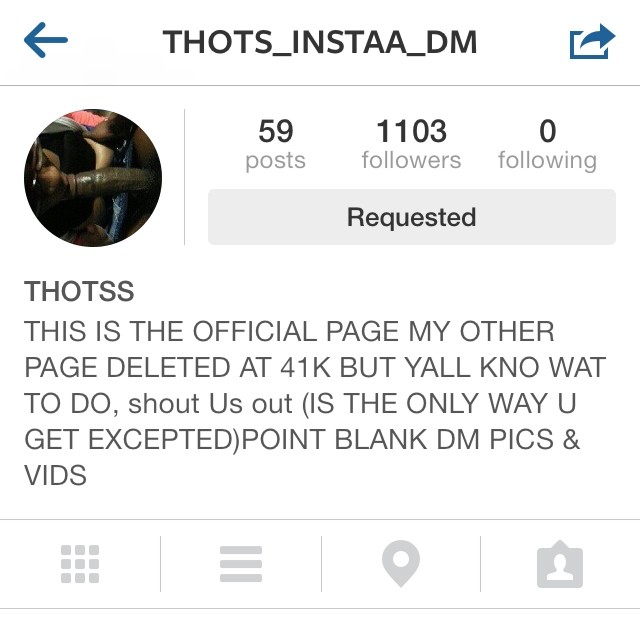The image is a screenshot of an Instagram profile for the user "thoughts_thotss," indicated by the Instagram handle "thoughts_insta_DM." The profile header includes 59 posts, 1,103 followers, and the account follows no one. A key detail is the status "Requested" shown on the profile, suggesting this is a private account. The bio reads: "This is the official page of my other page deleted at 41k, but y'all know what to do, shout us out (the only way you get accepted) point blank. DM pics and vids." The profile picture is unclear, but suggests inappropriate or explicit content. Above the bio, there is a blue back arrow on the top left, and a blue share button on the right, standard for Instagram interface. Additional interface elements like a grayed-out "Requested" button and various function buttons are also visible.